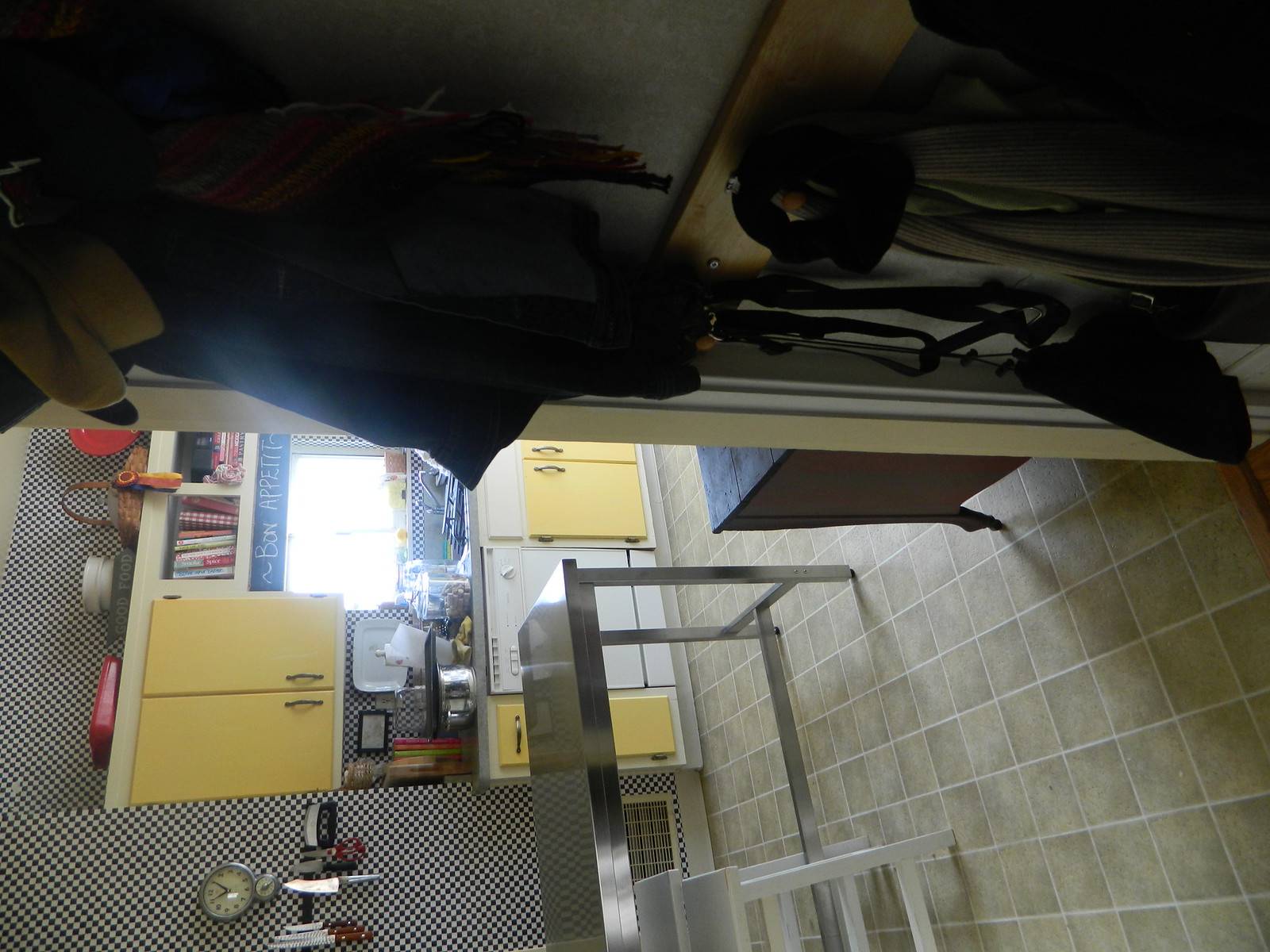The photograph captures a quaint kitchen viewed from the adjacent coat or entrance room, but appears rotated 90 degrees. The kitchen features a distinctive checkered wallpaper that adds a touch of vintage charm. At the center of the image stands a steel countertop, slightly cluttered with various kitchen items, reflecting a lived-in and practical space.

The upper and lower cabinets are painted a cheerful yellow, setting a bright and welcoming tone for the kitchen. The area above these cabinets is adorned with baskets and containers, offering both decorative and storage solutions. Antique white coloring forms the base and backdrop of these cabinets, balancing the vibrant yellow with a subtle, timeless contrast.

Natural daylight filters through a window positioned above the kitchen, illuminating the space with a soft, inviting glow. The floor is covered in vinyl, a practical choice likely intended for easy maintenance.

On the wall, a clock is mounted just above a magnetic strip holding an assortment of steak and cutting knives, emphasizing the kitchen’s functionality. Overall, this cozy and colorful kitchen scene reflects a blend of aesthetic appeal and real-world utility.